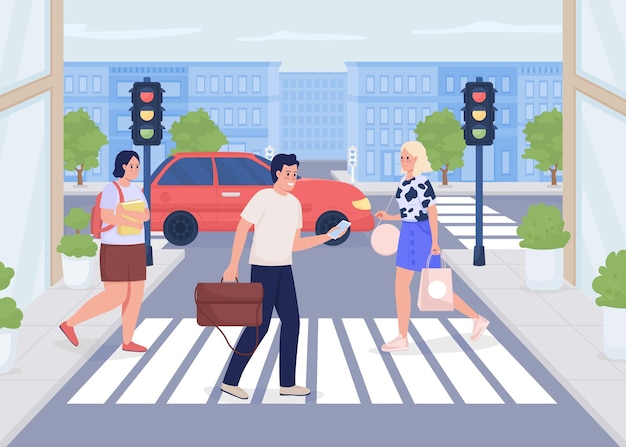A detailed, stylized, two-dimensional graphic image depicts a typical, bustling city street scene in the United States, filled with dynamic urban life and vibrant interactions. Three happy pedestrians are walking across a zebra crosswalk at a T-intersection, all dressed casually. At the center, a man in an ivory t-shirt, navy blue pants, and carrying a briefcase looks attentively at his phone, suggesting he might be on his way to work. Slightly behind him, on his right, is a black-haired woman in a light blue t-shirt, brown skirt, and red shoes, carrying a backpack and a book, hinting she is a student on her way to school. To the man's left, a blonde woman walks in the opposite direction, wearing a bright blue skirt and a distinctive white and black patterned blouse that resembles cow print, carrying a purse and a shopping bag, indicating she has been shopping.

The background is adorned with city street buildings, including brownstones and blue-toned apartment and office buildings. The scene captures a sunny day with no trash littering the clean sidewalks. There are stoplights at the corners of the intersection, and a red car is seen driving through the perpendicular street. Behind the crosswalk, trees add a touch of greenery, enhancing the visual appeal of this neat-looking cityscape. The image encapsulates the everyday hustle and bustle of city life, with everyone seemingly in a hurry, going about their daily routines.